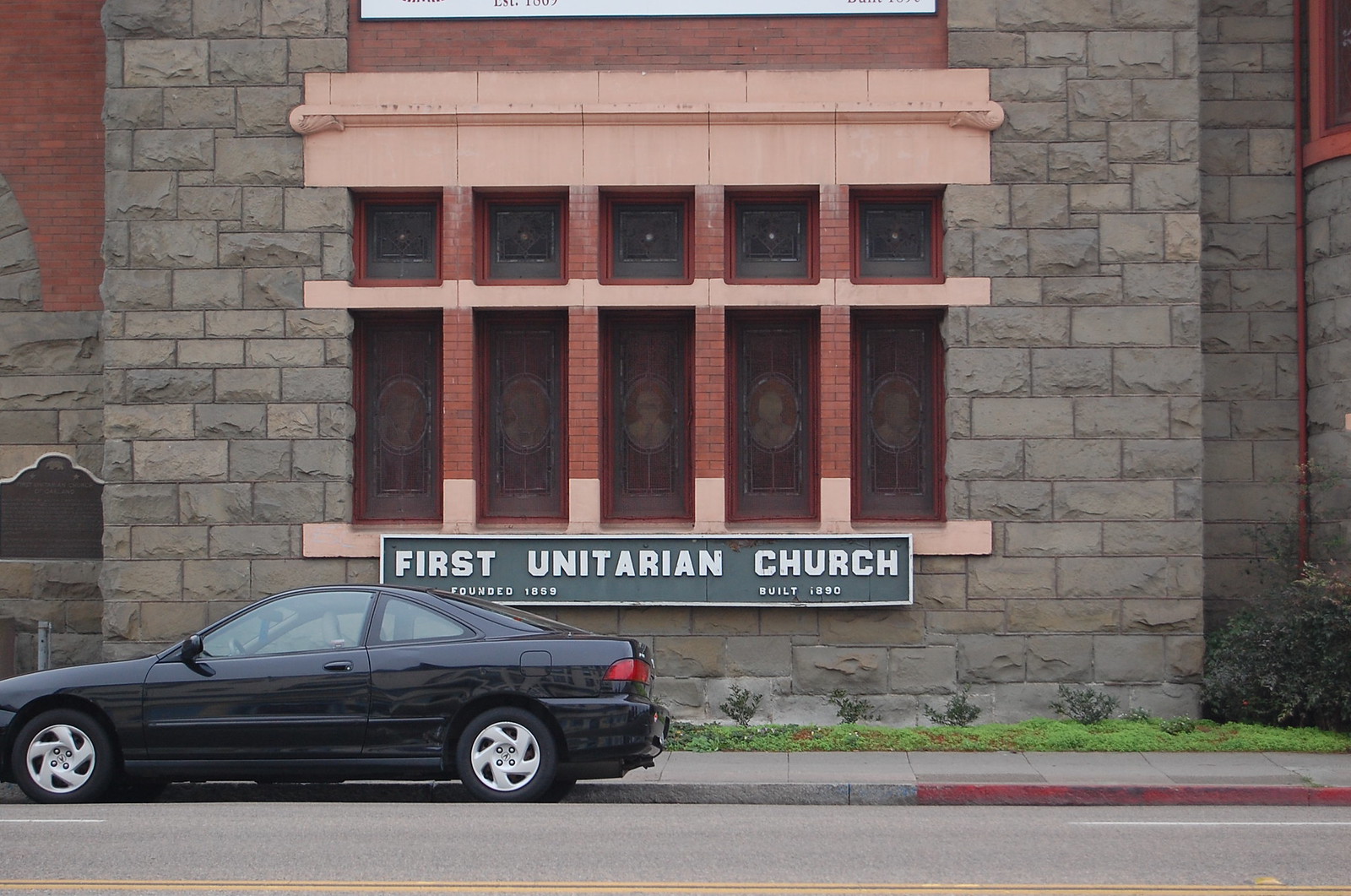A detailed image shows a modern black two-door Acura sedan with gray hubcaps parked alongside a gray sidewalk marked with a red stripe. The car is positioned in front of the First Unitarian Church, which is an impressive structure predominantly composed of gray rectangular stones, accentuated by red bricks framing the windows and sections of its foundation. This historic church, established in 1859 and constructed in 1890, prominently features a green plaque with white text denoting its name and foundation details.

The facade of the church displays a sequence of five large rectangular stained glass windows, each topped by smaller square panes. The stained glass, richly colored in maroon, black, and gray, depicts images of people and is bordered with brick accents. At the church’s base, there's an area of well-maintained green grass and darker green shrubbery. The photo, taken in the daytime, captures additional architectural details such as the pink sections of the foundation and an orange-tinted top window. The scene is set against the backdrop of a regular gray road, adding to the urban charm of this historical site.